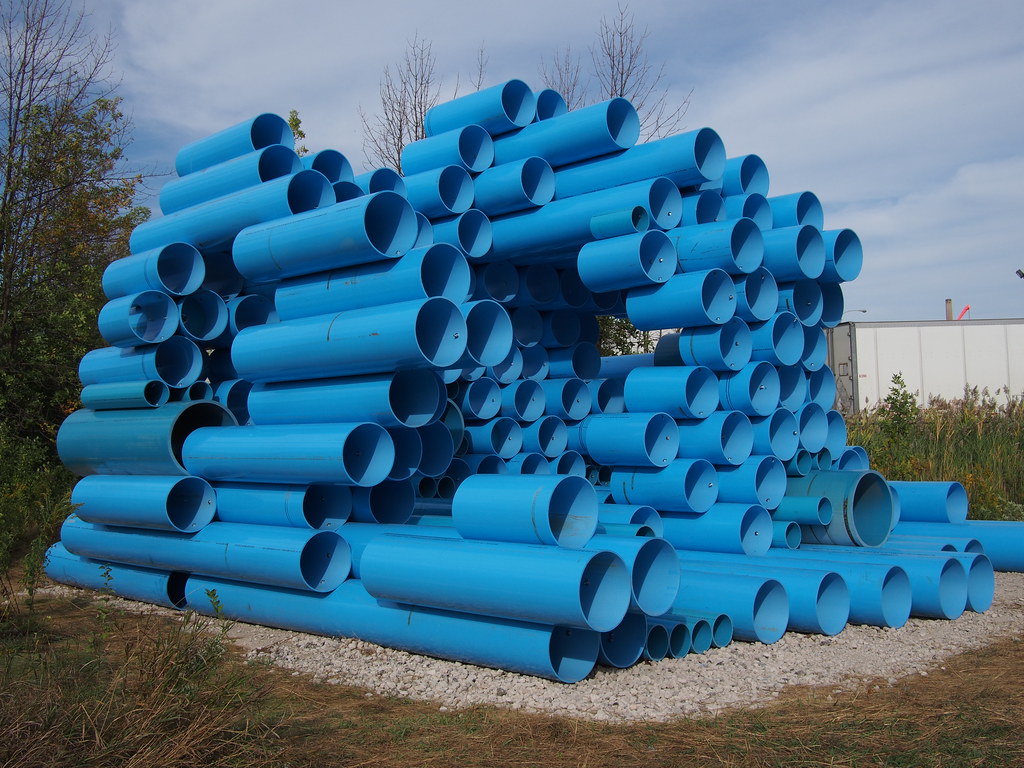In an outdoor daytime setting with a backdrop of a partly cloudy, blue sky, a striking sculpture made of turquoise blue tubes stands prominently at the center. These tubes, possibly numbering around 100, vary in length and diameter and are meticulously arranged in an artistic formation. The tubes are fastened to one another with visible metal objects on their insides, creating a sturdy structure that extends upwards in multiple layers. The entire assembly rests on a small bed of rocks, adding a textured base to the platform. Surrounding this rocky base, a patch of brownish-green grass, some of which appears to be dead, contrasts with the vibrant blue of the tubes. In the background, there are several tall, thin trees with sparse branches. Some branches bear light green and orange leaves, while others are bare, adding an element of natural beauty to the scene.